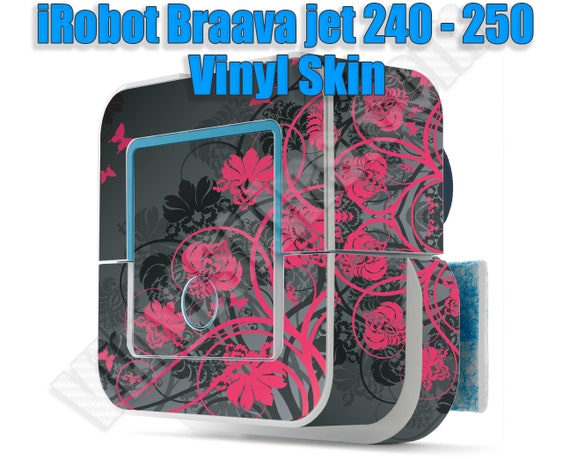The image is an advertisement for the iRobot Braava Jet 240-250 Vinyl Skin. It features a vibrant, specialized cover designed to give the iRobot a more customized appearance. The background is white, and at the top, the text "iRobot Braava Jet 240-250 Vinyl Skin" is prominently displayed in blue font.

The vinyl skin itself, showcased in the image, has a predominantly gray background with a striking design of pink and red flowers and curved pink lines spread across it. There are also red butterflies carefully placed in the top left corner of the device. This skin gives the iRobot a distinctive black and red color scheme. The device, which resembles a vacuum robot, is partially visible from an angled perspective, revealing a large front button with a blue circle and blue square on the side, as well as a piece of blue and white material sticking out from behind it. The overall design aims to enhance the aesthetic appeal of the iRobot while maintaining its functional aspects.